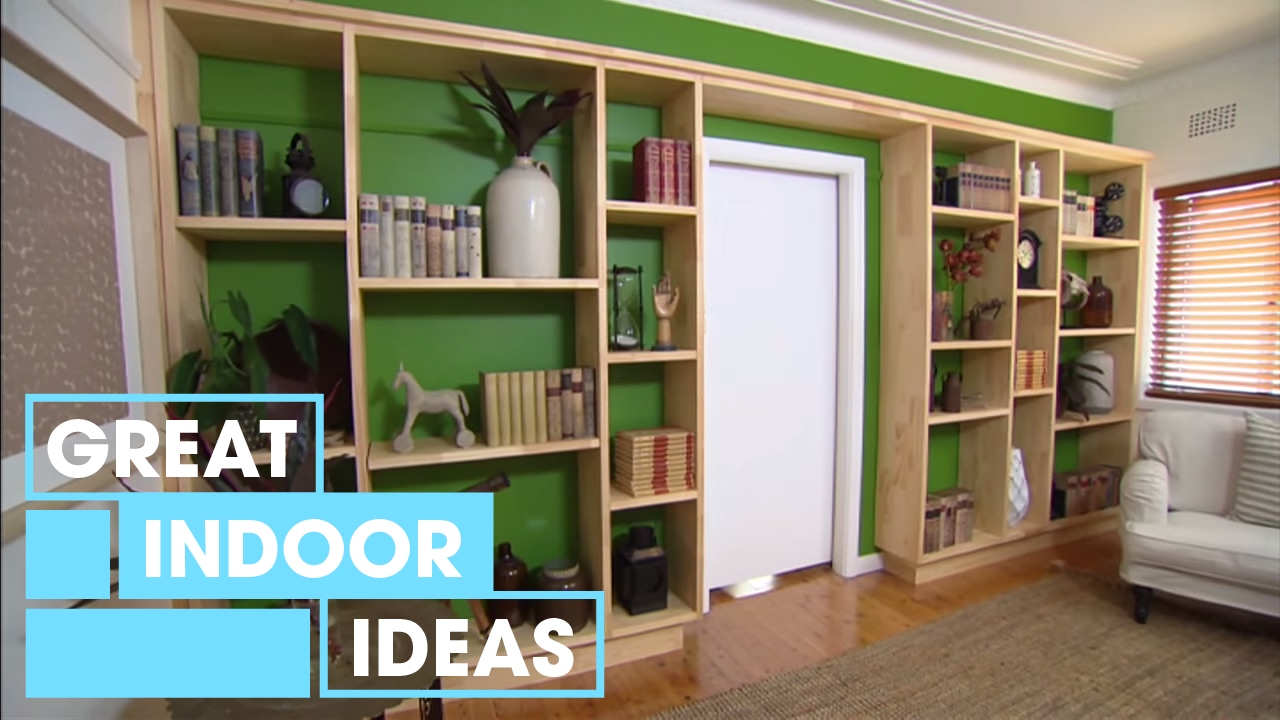This image is an advertisement for interior design, showcasing a meticulously organized room with detailed decor. The focal point is a floor-to-ceiling bookcase constructed from light pine, seamlessly built into a bright green wall adorned with white molding near the ceiling. The bookcase, divided into two sections by a central white door framed with white trim, is filled with an assortment of books, figurines, vases with plants, and various decorations including a clock and a small horse sign. Beneath the bookcase, the room features a light hardwood floor partially covered by a tan rug that bears the phrase "great indoor ideas." A cream-colored couch is situated on this rug, positioned in front of a window equipped with closed blinds. The room's inviting atmosphere is completed with the presence of smaller design elements such as knickknacks and flowers, contributing to a coherent and charming aesthetic.